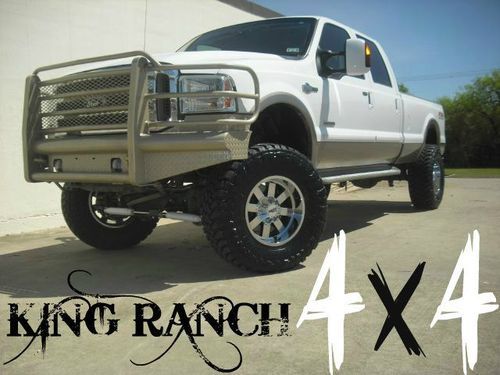The image features a large white Ford pickup truck prominently positioned in the middle of a road. The truck, which appears to be a King Ranch 4x4 model, boasts wide black tires and a distinct two-tone color scheme, with a white upper body and a beige lower trim. Notably, the truck has an added beige-colored graded bar covering the grill and headlights, enhancing its rugged appearance. This bar extends over the front grill, adding a layer of protection. The truck is a four-door model with wide mirrors, and the driver's side is particularly visible. It sits higher off the ground, indicative of its robust build and large wheels. In the background, to the left of the truck, is a building, while to the right are lush green trees. The sky is a clear blue, suggesting a bright and sunny day. Written at the bottom of the image are the words "King Ranch 4x4," with "King Ranch" in black letters, and the numbers "4" in white letters flanking a black "X." The truck's lights seem to be on, but there is no visible occupant inside.